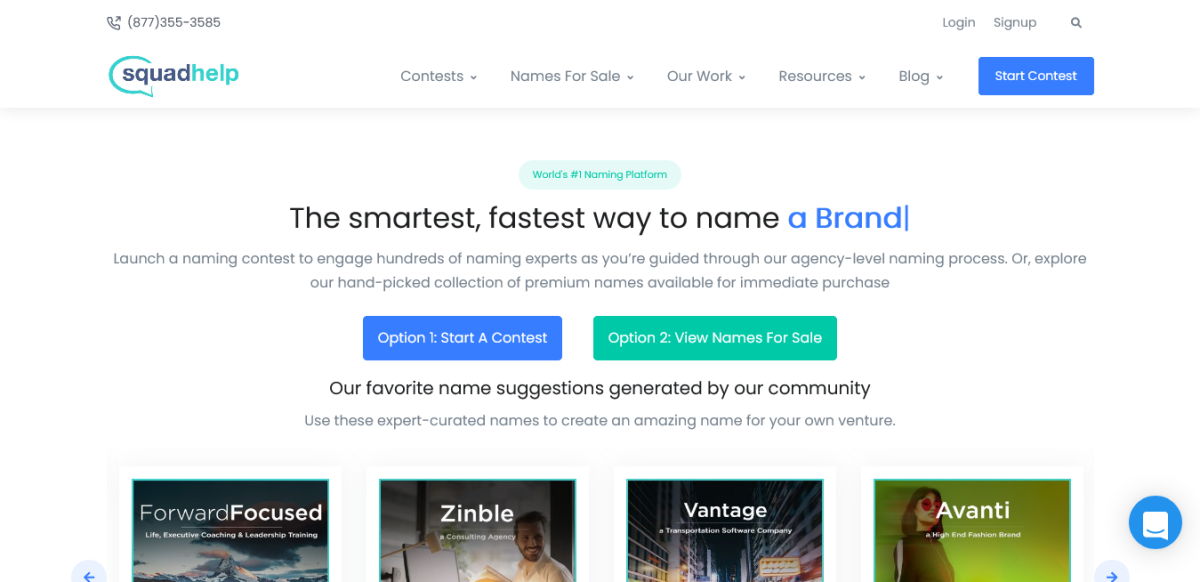The image is a screenshot from a website, meticulously detailing its layout and functional elements. In the top left corner, there is a prominently displayed phone number, 877-355-3585. On the top right corner, options for "Log In," "Sign Up," and a search icon are visible.

Aligned to the left is the Squad Help logo, followed by a series of pull-down menus labeled "Contests," "Names for Sale," "Our Work," "Resources," and "Blog." Adjacent to these menus, on the right side, is a blue rectangle button labeled "Start Contest."

The main content of the webpage is set against a white background. At the top, there's a pale green oval containing green text that proclaims "World's Number One Naming Platform." Beneath this, black text declares, "The Smartest, Fastest Way to Name," followed by blue text, "A Brand." In gray text below, it explains, "Launch a Naming Contest to Engage Hundreds of Naming Experts as You're Guided Through Our Agency-Level Naming Process, or Explore Our Handpicked Collection of Premium Names Available for Immediate Purchase."

Two rectangular buttons are below this description: a blue one labeled "Option 1: Start a Contest," and a green one labeled "Option 2: View Names for Sale."

Further down, black text introduces "Our Favorite Name Suggestions Generated by Our Community. Use these expert curated names to create an amazing name for your own venture." Below this statement, a row of four photographs features names like "Forward Focused," "Zimble" (spelled Z-I-N-B-L-E), "Vantage," and "Avanti" (spelled A-V-A-N-T-I).

Finally, on the bottom right corner of the screen, a blue circle displays a chat logo, indicating a chat support option.